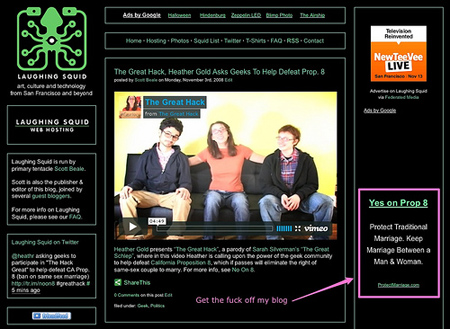This screenshot, taken from the website Laughing Squid, features a predominantly black background. The upper left corner displays the website's name, "Laughing Squid," in white font alongside an icon of a golden squid. Below the site's name, the text reads, "Art, culture, and technology from San Francisco and beyond.”

Further down, it mentions that "Laughing Squid is run by primary tentacle Scott Beale. Scott is also the publisher and editor of this blog, joined by several guest bloggers. For more info on Laughing Squid, please see our FAQ."

In the center of the webpage, there is a prominent Vimeo video link labeled "The Great Hack." The video preview shows three young adults, likely in their early 20s, all wearing glasses and sitting on a couch. A girl sits in the middle, flanked by two guys on each side. 

Additionally, someone has altered this screenshot by adding a small arrow and comment, but the details of this annotation are unclear. The rest of the text on the page is densely packed and challenging to read.